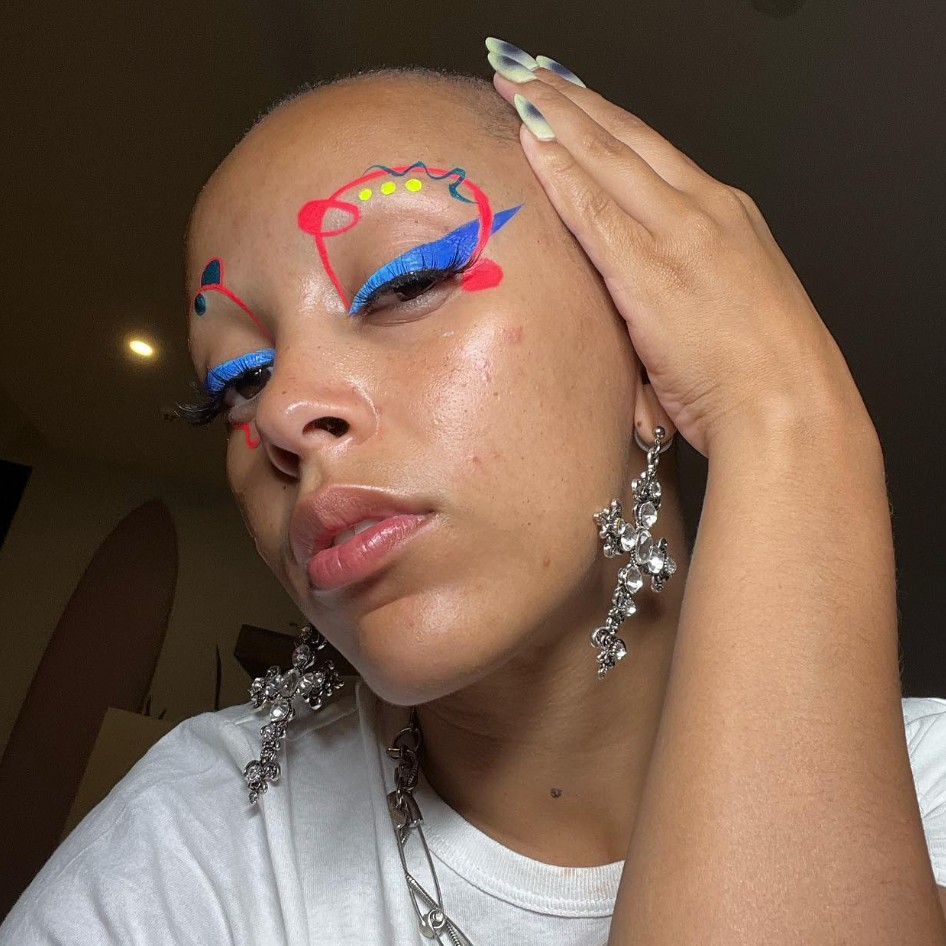In this close-up image, Doja Cat showcases her elaborate and artistic makeup. She wears a simple white t-shirt, with a unique safety pin necklace and large silver and clear crystal cross dangly earrings. Her short hair is shaved, revealing her bold makeup design. The makeup features exaggerated eye details, including elongated cat-eye eyeliner that transitions from light blue at the inner corners to a deep blue wing. Above each eye is a red three-quarter circle, with her left eye adorned with three yellow dots and a superimposed blue squiggly line, while her right eye has a blue dot inside the circle. Her hand, delicately placed against her tilted head, displays long fake nails painted a yellowish-cream color with a dark bluish-gray center, resembling a solar eclipse. The background is mostly dark with a recessed light visible behind her, giving a striking contrast to her vivid makeup.